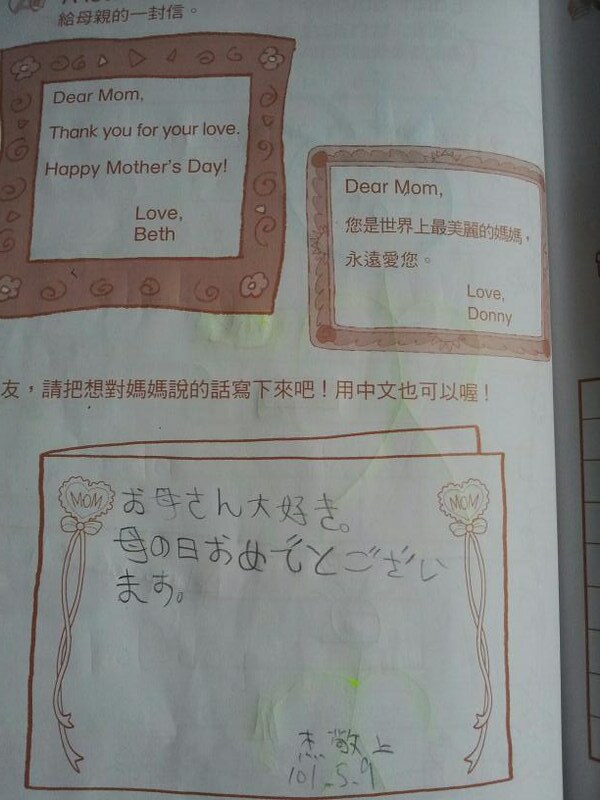This image features a piece of paper with a white background, decorated with various heartfelt texts and designs. At the top left, there is a brownish-red bordered box adorned with flowers and swirly lines. Inside this box, written in the same brownish-red color, is the message: "Dear Mom, thank you for your love. Happy Mother's Day. Love, Beth." To the right of this, there is a smaller, similarly decorated box. It contains the text, "Dear Mom," followed by phrases in Mandarin or possibly Kanji, and concludes with, "Love, Donny." Below these two main boxes, there is a line of additional text in Mandarin or Kanji, followed by an outline drawing of a card. This card features hearts in the upper corners and ribbons stating "Mom" on the right and left sides, with more text in the same foreign script. The image has green stains, indicating it is likely a children's creation. At the very bottom, the numbers "101.5.9" are written.